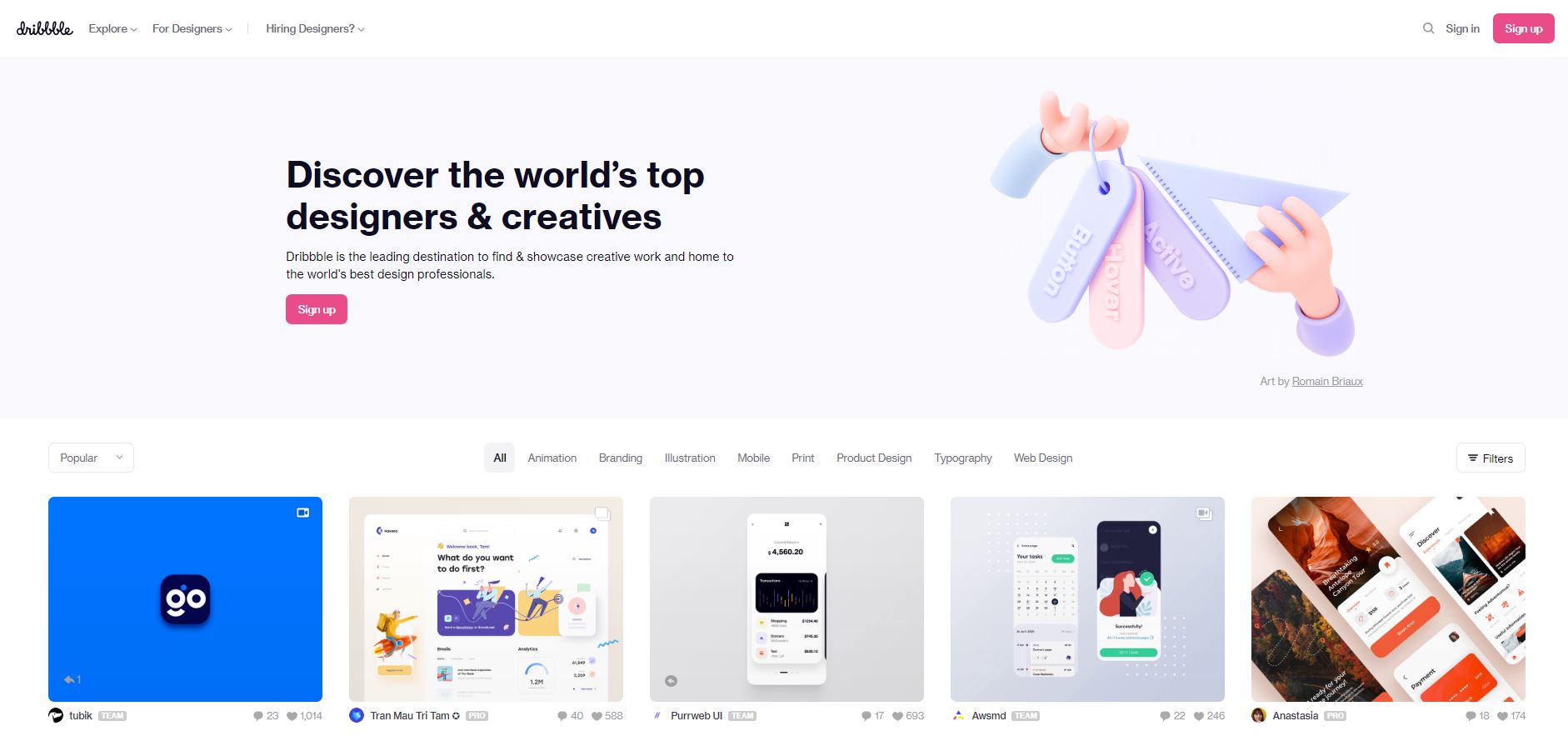This image depicts a computer screen displaying a webpage from Dribbble, a popular platform for designers. At the top of the screen, the Dribbble logo is prominently displayed in black cursive text, spelled "D-R-I-B-B-B-L-E." Next to the logo are navigation links labeled "Explore," "For Designers," and a banner with the text "Hiring Designers?" 

Centrally positioned in the image are a pair of hands holding a key ring, which has tags labeled "Active," "Button," and "Hover." Additionally, a math utensil is held between the fingers, suggesting the precision and creativity in design work. Above this central image is the headline "Discover the World's Top Designers and Creatives."

Below this, the site description reads: "Dribbble is the leading destination to find and showcase creative work and home to the world's best design professionals." A prominent pink sign-up button is positioned nearby, encouraging new users to join the platform.

Towards the bottom of the screen, several clickable areas feature thumbnail images, providing additional navigation options for exploring more content on the site.